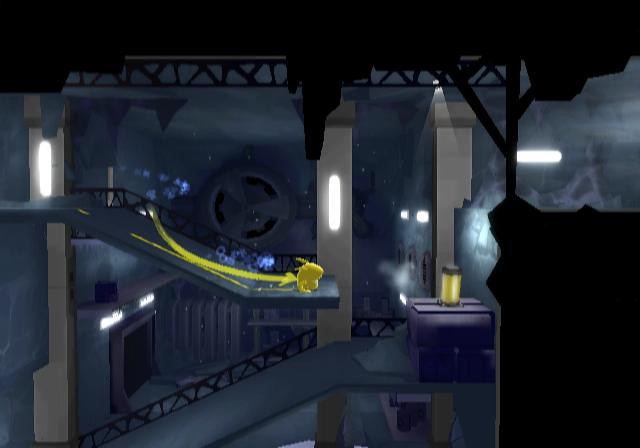The image appears to be a vivid frame from a video game. Central to the scene is a small, yellow creature that closely resembles Pikachu, standing poised at the edge of a broken bridge. The character seems readying for a daring leap towards a glowing yellow canister, potentially a life-extending bonus. A curved yellow arrow directs the creature's path, emphasizing the dynamic moment. Surrounding this action are grey pillars equipped with white fluorescent lamps jutting from their sides, suggesting an industrial setting. In the background, a dark, greyish cavern adds a sense of depth and mystery, solidifying the impression that the creature is navigating through a complex factory or facility.